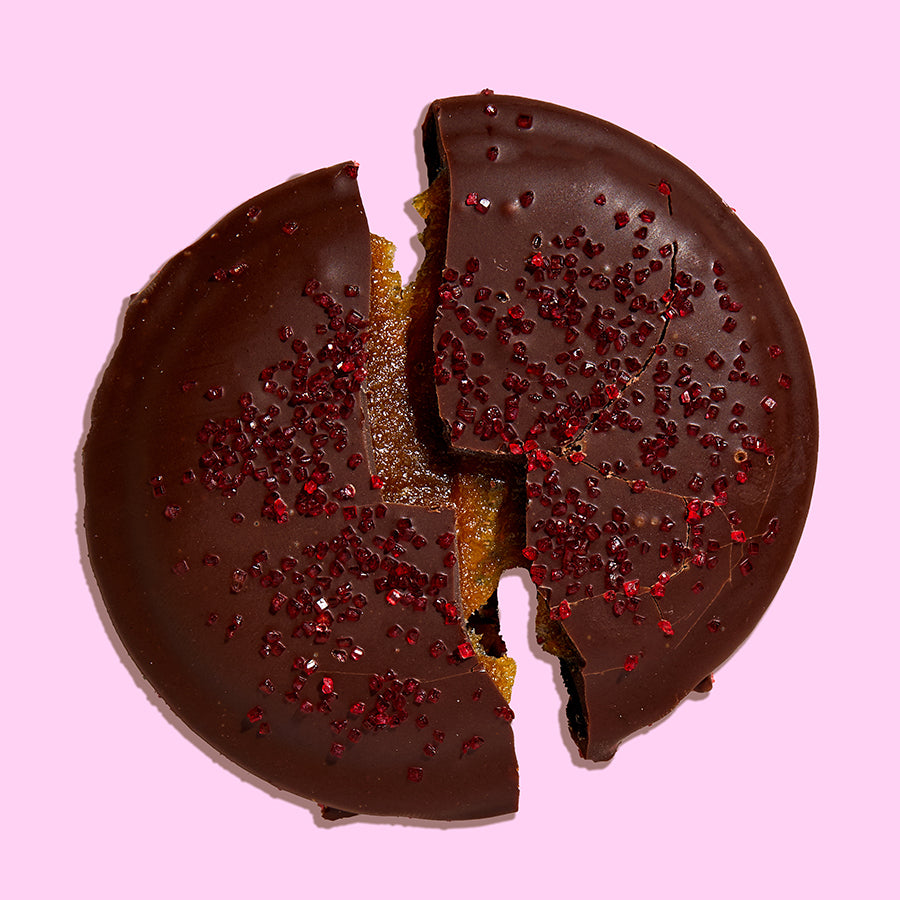The realistic photograph features a round, disc-shaped chocolate cookie placed against a square-shaped pink background. The cookie, primarily brown in color, is split in half, revealing a jam or jelly filling inside. The filling appears tan to orange in hue, possibly suggesting apricot or orange flavor, and has a glossy, sugary texture reminiscent of a custard or a sugar glaze. The top of the cookie is adorned with small, red, candy-like sprinkles or rocks. The image is highly detailed and zoomed in, with the cookie centered and occupying the majority of the frame, emphasizing its detailed textures and colors.